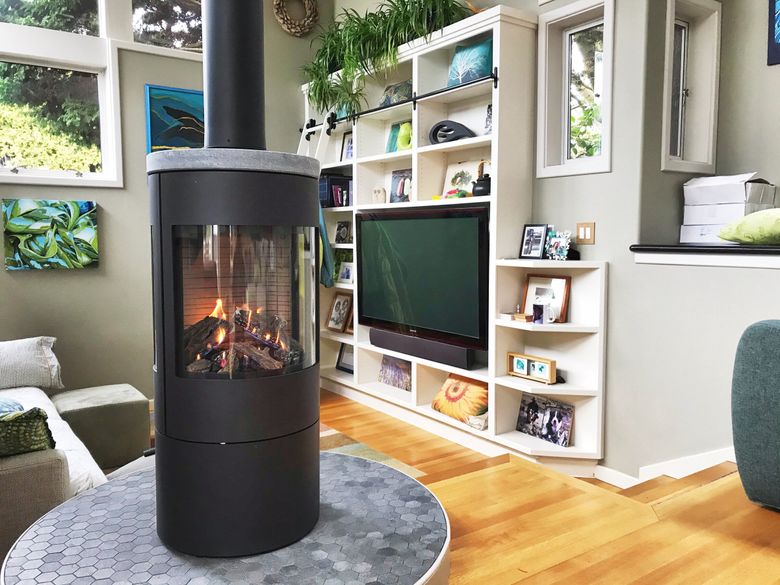The image depicts a cozy living room with a variety of detailed elements. Central to the room is an enclosed, cylindrical fireplace with a fire burning inside, placed atop a gray mat featuring hexagonal patterns. Surrounding the fireplace is a wooden floor. To the right, part of a dark gray furniture piece is visible, adorned with three white objects. On the left side, the arm of a tan-colored couch can be seen, and a white section of a sofa. Shelving units with four columns occupy the center portion of the image, housing a flat-screen TV and various items, including pictures, pillows, and houseplants with lush green foliage. Atop the shelves are several decorative houseplants. The walls are adorned with various framed artworks and decorations, including paintings in blue and green hues and a circular or oval brown object. A window situated in the top left corner offers a view of green foliage outside, enhancing the room's inviting ambiance.